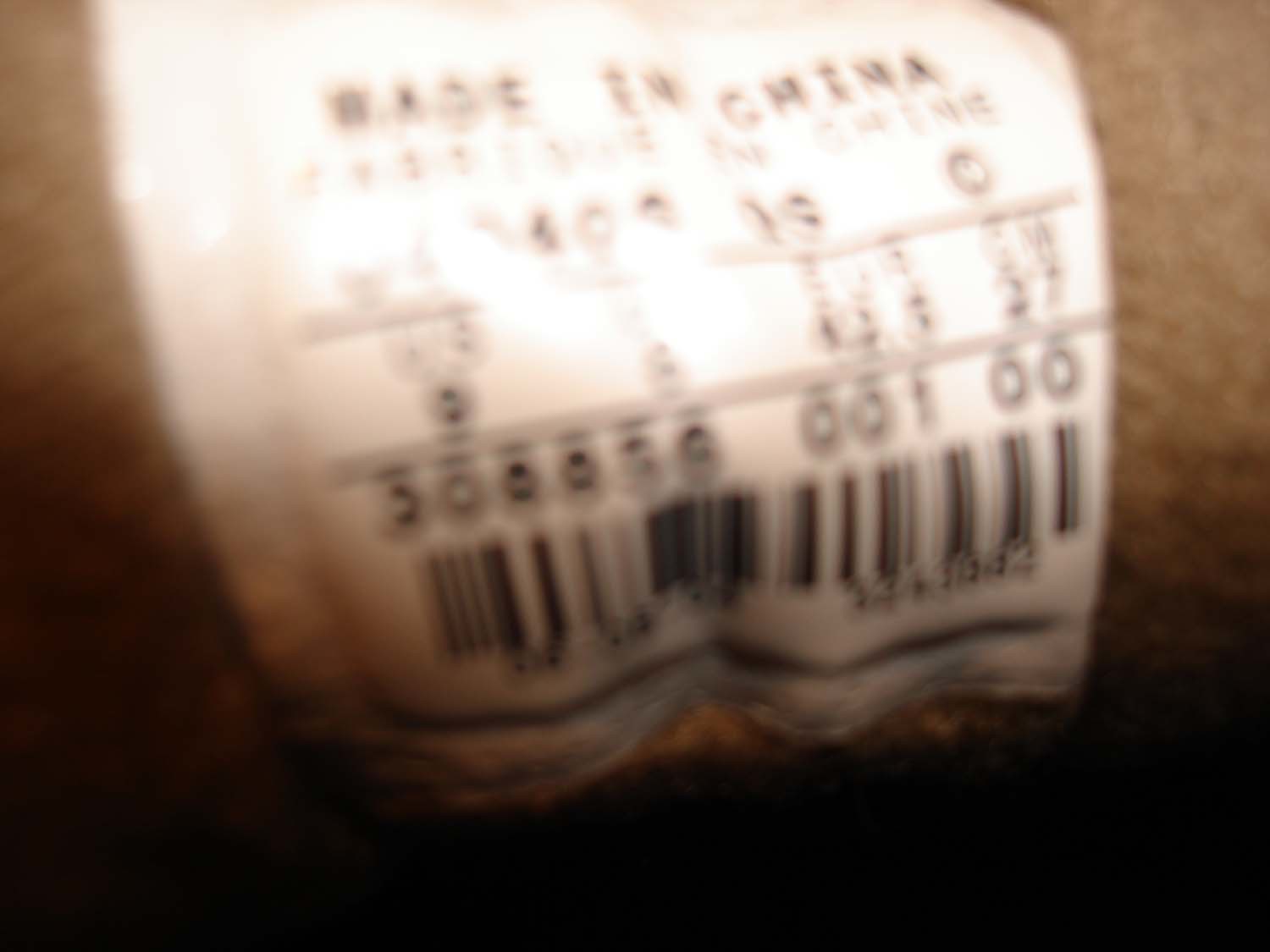The photograph is a close-up, albeit a highly blurry one, of a white label or tag. The tag is affixed to a curved object, which remains unidentified due to the zoom and angle of the shot. Prominently, at the top of the tag, in bold black lettering, it reads "Made in China." Below this phrase, there are several rows of black characters and numbers, which are mostly illegible except for a few discernible digits: 8, 5, 6, 0, 0, 1, 0, 0. These numbers might represent a serial number or possibly shoe sizes, though it's too blurry to confirm. Toward the bottom of the tag is a black and white barcode. The background of the image appears to be a blurry, tan surface, which could be carpet or another textured material. The tag itself seems to be draped over or attached to a medium cocoa brown object, possibly gathered or slightly folded, adding to the difficulty in identifying the exact nature of the item it is labeling.